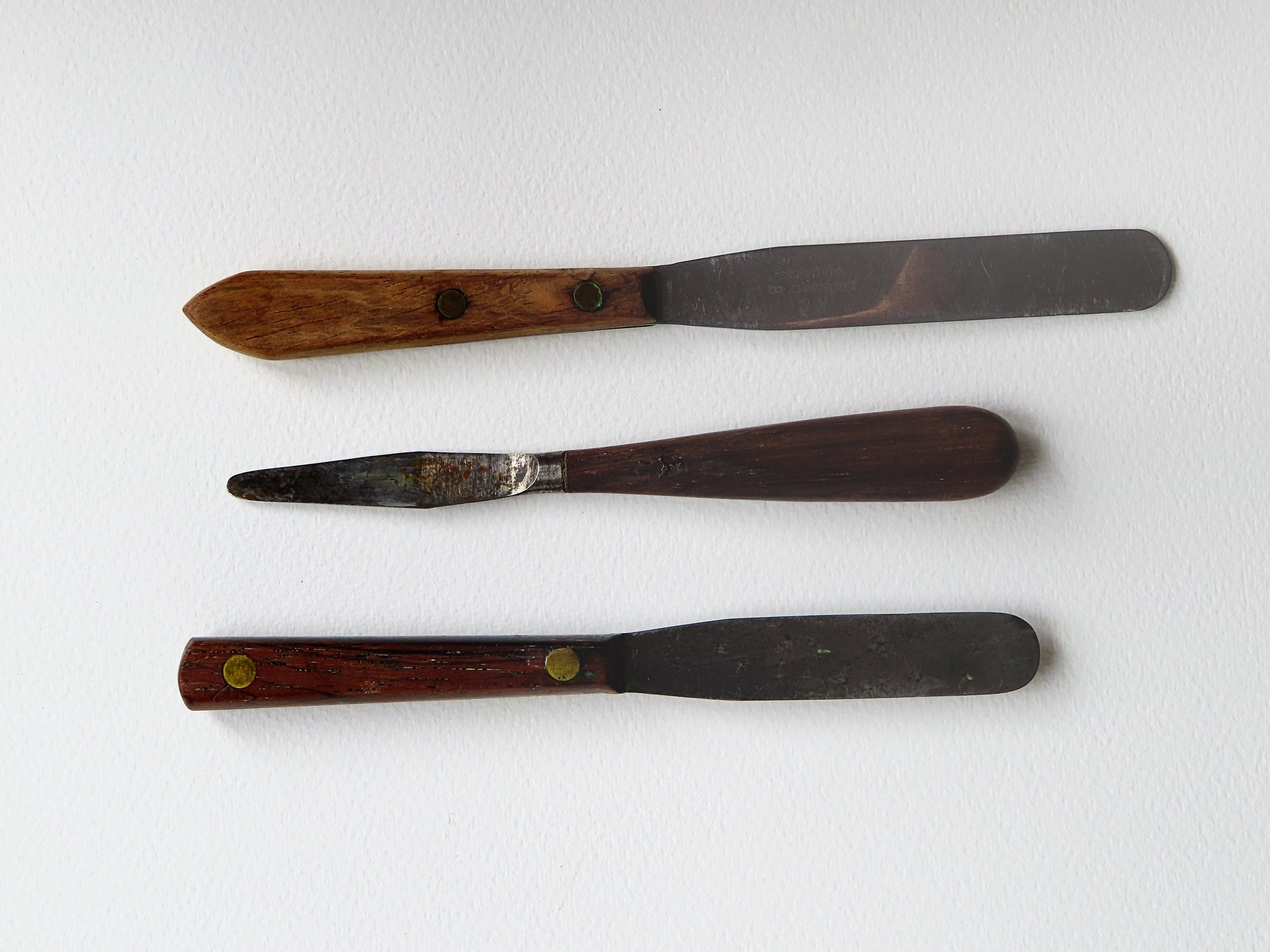On a rectangular photograph taken indoors, resting horizontally on a light gray or off-white textured tabletop, three antique woodworking tools are meticulously displayed. At the top lies a long, dark gray metal tool resembling a nail file, featuring a light walnut-colored wooden handle secured with two round bolts. The tool directly below has a thicker, dark brown wooden handle, with a blade that widens at the center and narrows at the tip, reminiscent of a scraper or scooper. The bottom tool, though smaller, mirrors a similar nail file form, possessing a dark wood handle adorned with two brass circles at the top and bottom, and a long, narrow metal blade with a rounded front. Each tool's metallic component and wooden handle are positioned oppositely for the top and bottom tools, while the middle tool's structure contrasts by reversing this order.